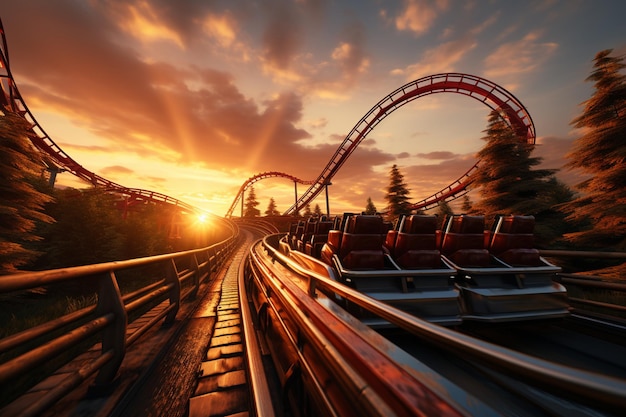In the artistic photograph taken at sunset, the rollercoaster track spirals dramatically against a partially cloudy sky colored in gradients of gray, blue, yellow, and orange. The track, resembling a snake, features high curves and significant loops on both sides, accentuating its wavy and elevated structure. Towards the right center of the image, an empty rollercoaster car painted red sits idle, its multiple rows of seats awaiting passengers. Evergreen pine trees are scattered across the scene, prominently visible on the right and center, blending into the distant background. The golden-yellow sun dominates the horizon, its rays streaking outward and reflecting off the clouds, creating a mesmerizing interplay of light and shadow that bathes the entire scene in a warm, serene glow.